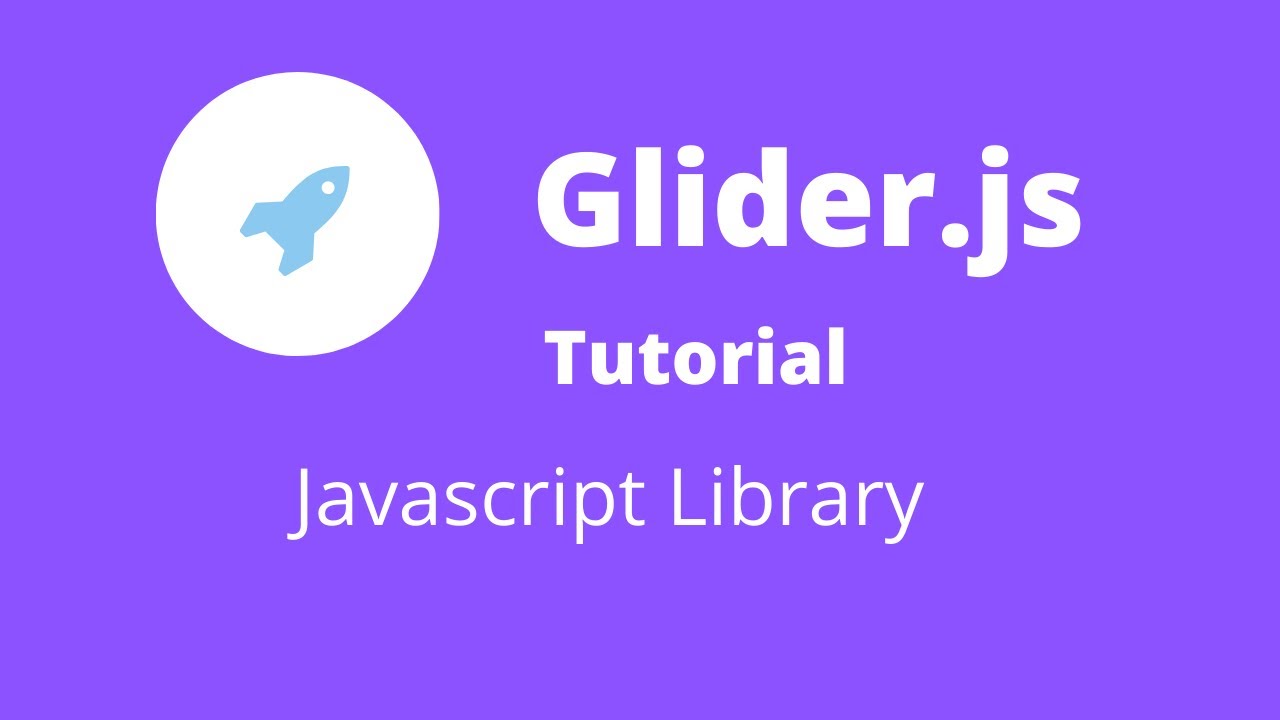The image showcases a rectangular tutorial banner dominated by a purple background. In the upper-left section of the rectangle, there is a white circle featuring a blue rocket, emphasizing the tutorial’s theme. Positioned to the right of the circle, the word "glider.js" is prominently displayed in a large, bold typeface, drawing immediate attention. Below "glider.js," the word "tutorial" appears in a slightly smaller but still noticeable font. Further down, the phrase "javascript library" is written in a notably slender text. The varying font weights—bold for "glider.js," medium for "tutorial," and light for "javascript library"—create a hierarchical visual arrangement, ensuring clarity and focus. Overall, the design elements are meticulously centered within the purple rectangle, accentuating the banner’s modern and organized look.